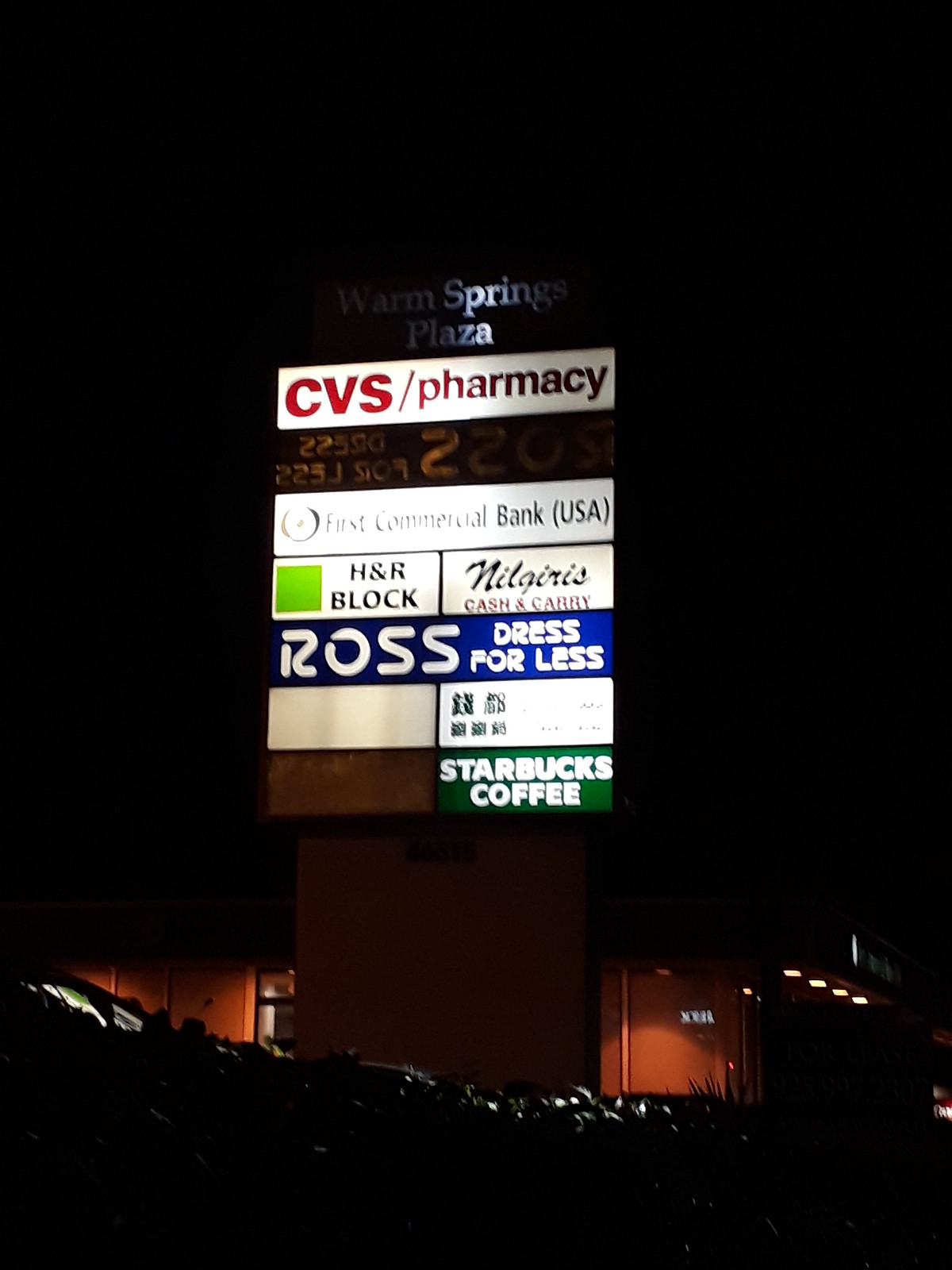A nighttime photograph captures the bustling shopping area of "Something Springs Plaza". Despite the darkness, the outlines of several parked cars are faintly visible. At the top display, prominently lit, the plaza’s name stands out. 

Key stores within the plaza include a CVS Pharmacy, recognizable by its red lettering on a white background. Adjacent to it is a First Commercial Bank, USA, distinguished by what appears to be a dark navy logo, complemented by "USA" in parentheses. 

Further down, the space is split between an H&R Block, notable for its green square logo, and "Nigeria's Cash and Carry," presumably a convenience store, marked by a blue sign with modern white fonts. Below them, a "Ross Dress for Less" sign stands out with its modern blue and white design, indicating a clothing retail store.

An empty storefront below is now out of business. On the right side, signs in an unfamiliar language suggest a potentially diverse commercial presence. Adjacent to it, the familiar logo of "Starbucks Coffee" is illuminated.

The plaza is well-lit, guiding visitors through its extent, though individual storefronts blend into the night, only the path beyond remaining visibly well-lit.